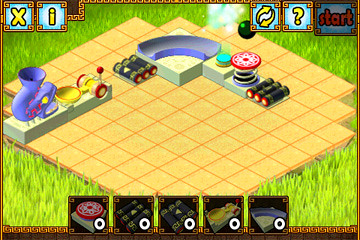This image is a detailed screenshot from a video game, prominently featuring a unique grid-based interface. The central element is a grid of yellow squares, forming a roughly 8 by 8 configuration with truncated corners. Interspersed across this grid are various objects: a quarter-circle figure, two clusters of three gray cylinders each laying on their sides resembling batteries, a large red and white button, a smaller aqua button, and a curved tube. Along the bottom of the screen, five additional squares display different components, currently indicating zero inventory. Above the grid, the interface includes functional icons: a yellow-lettered "X" and "I" within squares, a pair of directional yellow arrows on a blue background, a yellow question mark on a blue background, and a "Start" button. The entire setup is reminiscent of a game board laid over green and yellow grass.